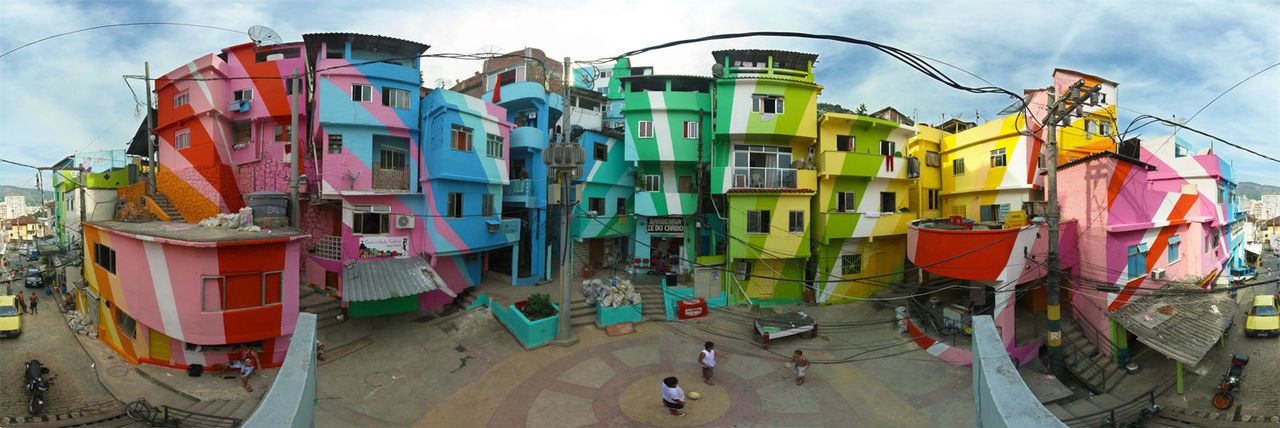The photo presents a vivid and colorful scene of an apartment complex, capturing a vibrant community under a clear blue sky dotted with white clouds. The buildings are painted in a striking array of colors resembling a rainbow, with each structure adorned with diagonal and horizontal stripes. The first building showcases a blend of red, blue, and pink, transitioning seamlessly into adjoining structures painted in blues, greens, and yellows, creating a visually engaging palette reminiscent of fruit-striped gum. Despite what appears to be a low-income neighborhood, where streets are littered with debris, the paint job breathes life and charm into the area. The complex, comprising three-story high blocks, features balconies and a set of steps leading up to the units. Children are seen playing, kicking a ball around, and at a distance, parked cars and a black motorcycle add to the bustle of the scene. A person in a red shirt sits nearby, contributing to the lively atmosphere of this picturesque urban enclave.